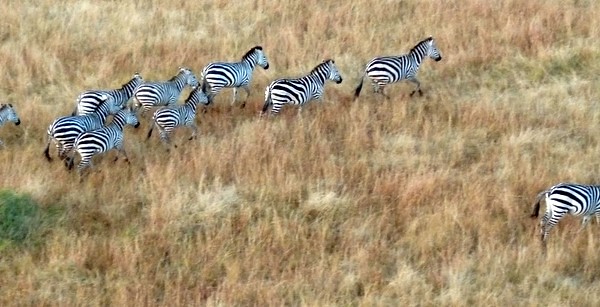This is a detailed landscape photograph of a herd of ten zebras traversing a grassland. The scene captures the animals moving from the left to the right across high, orangey-brown, and beige grass that appears slightly dried out. A touch of green vegetation is notable in the lower left corner of the image. The zebras are distinguished by their iconic black and white stripes.

Eight zebras form a clustered group, running in a diagonal line from the upper left to the center of the image. One zebra's head is just coming into frame from the left, and another zebra, located at the lower right, is slightly apart from the group, with only its back half visible as it exits the frame. The zebras appear to be commuting at a steady pace, giving the impression of movement across their natural habitat. This detailed composition offers a dynamic glimpse into the lives of these majestic animals as they navigate the grassland.